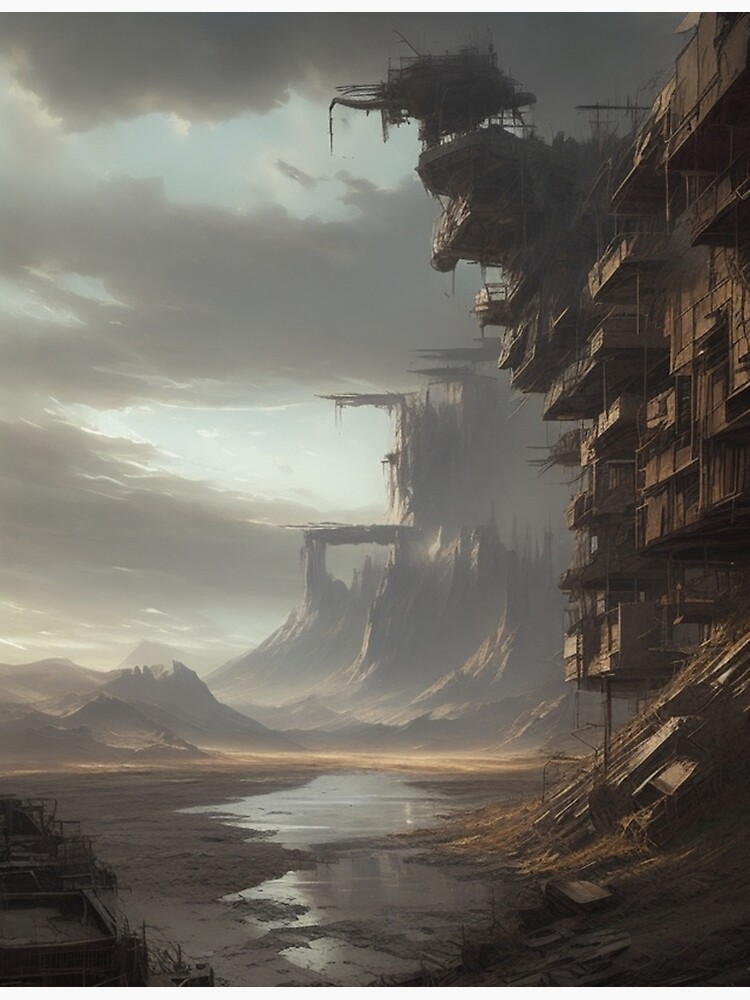The image is an artistic, possibly AI-generated drawing of a desolate, desert-like landscape, evoking a sense of gloom and destruction. The foreground features numerous ruined buildings, some appearing to have been left incomplete and subsequently ravaged by time, weather, or even conflict, suggesting severe damage akin to a dystopian setting. These structures, potentially made of wood, exhibit signs of collapse and erosion, with much more rubble concentrated on the left side. The ground is muddy and contains reflective puddles that mirror the dim and dark clouds overhead, indicating a presence of water amidst the dirt. In the background, there are pointed, spiky mountains under a sky heavy with dim, dark clouds, contributing to the eerie and foreboding atmosphere. Another structure can be seen in the distance, further enhancing the sense of widespread devastation and the absence of life.